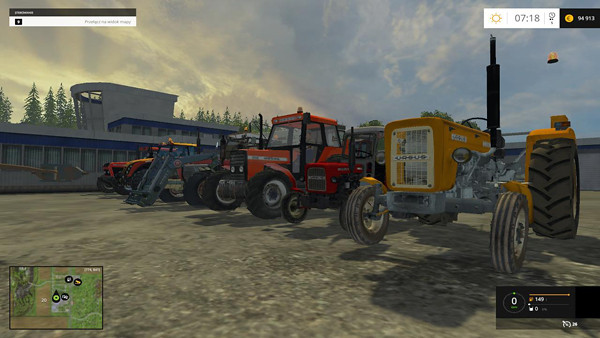This detailed horizontal, rectangular color photograph appears to be a screenshot from a video game, capturing a lineup of various tractors. Centered in the image are multiple tractors in different colors and shapes. The lineup includes vibrant yellow, red, and orange tractors, with the closest yellow tractor featuring a unique front opening, possibly an entrance. The red tractor in the middle has a conventional door similar to a car, while the orange tractor on the far left includes a silver ladder at its base.

To the left of the tractors, there's a modern building, reminiscent of an airport structure, with gray walls and blue trim. Towering pine trees stand behind the building, enhancing the scene's natural surroundings. The sky above is dramatic, displaying a mix of light, stripy clouds, and patches of blue sky.

The image includes various on-screen elements typical of a video game interface. In the upper right corner, the temperature and time are displayed, while a black circle with a white zero appears in the lower right corner. The upper left corner features a thin rectangular strip with a black top half and a white bottom half. Additionally, a map or grid with green and brown areas, indicating the player's location in the game, is positioned in the lower left corner.

Overall, the composition, vibrant colors, and interface details suggest that this is an AI-generated or digitally-rendered screenshot from a video game.